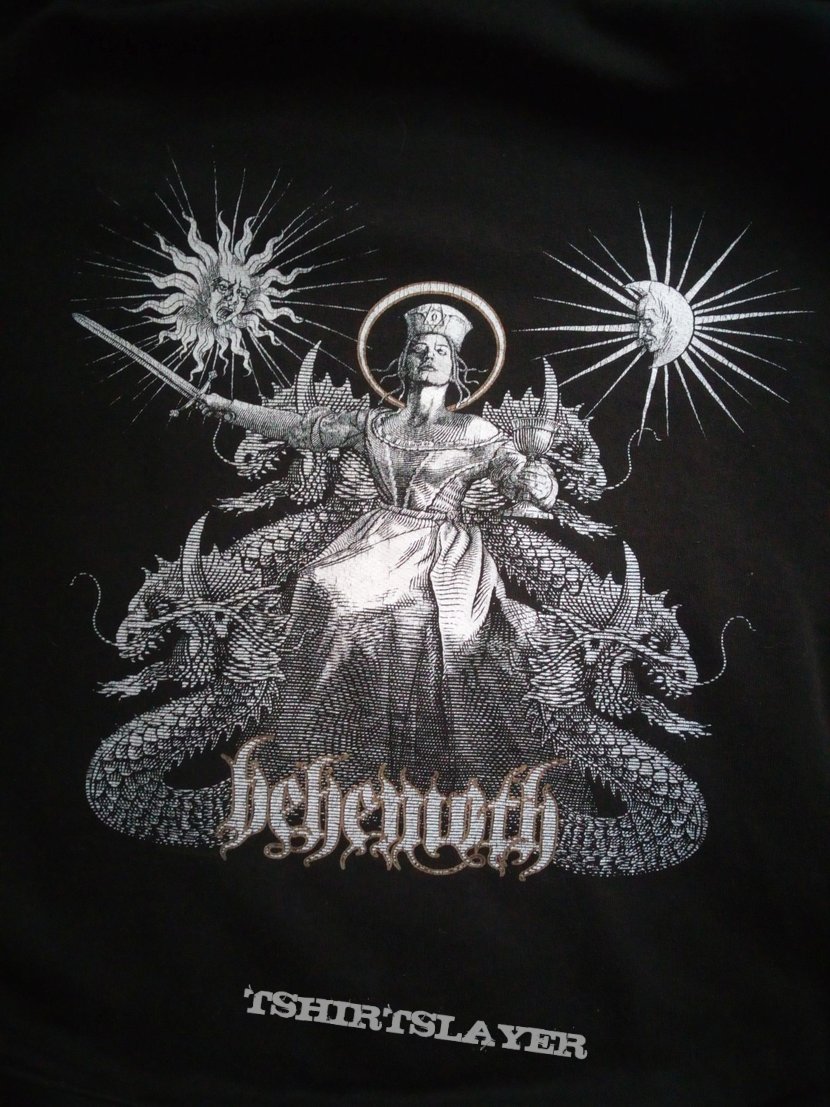In the image, a detailed grayscale graphic is set against a black background. Central to the composition is a woman adorned in medieval-style clothing, including a crown-like hat with a halo around her head. She stands poised with a sword in her right hand and a chalice in her left. Surrounding her are four dragon heads: two emerging from her shoulders and two flanking her hips, with their sinuous bodies coiling around her feet. The scene is further embellished by a personified sun on her left and a personified moon on her right, both radiating with pointed rays. Below her, the word "Behemoth" is prominently displayed in gothic stylized text, flanked by two more serpents. At the very bottom, the graphic is labeled “T-Shirt Slayer,” suggesting it could be a design intended for apparel. The overall aesthetic is both mythological and ornate, rendered primarily in silver and white tones, enhancing its medieval and mystical aura.